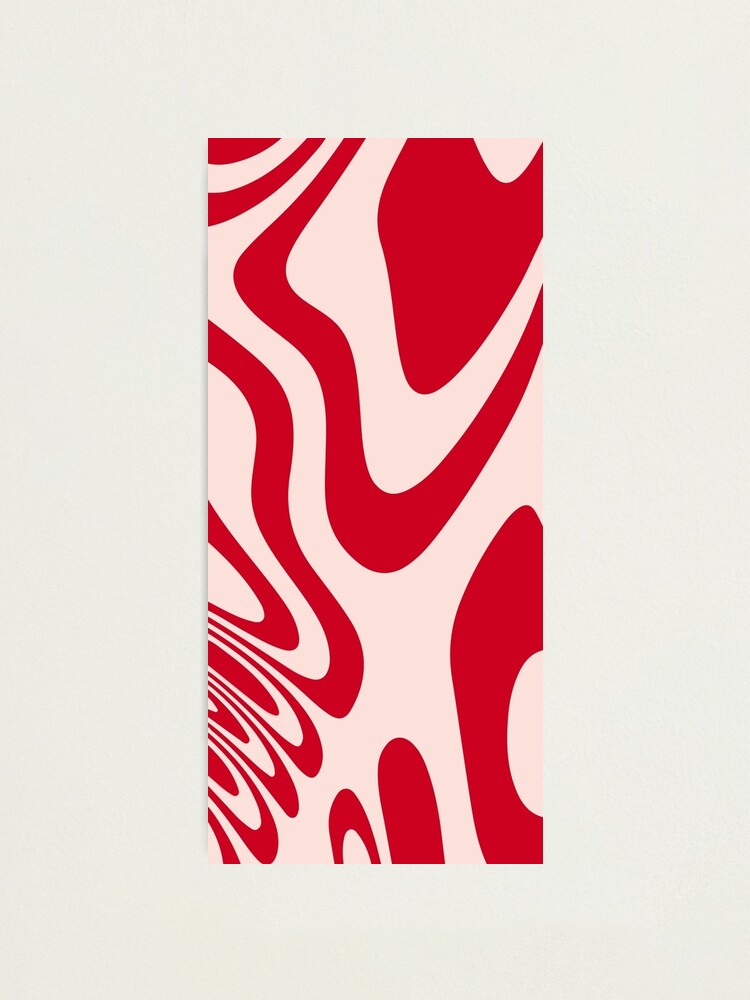This image features a rectangular artwork against a neutral white background. The artwork itself is characterized by bold, wavy red lines and large red blots set against a pink backdrop, giving it a surreal, almost Dali-esque quality. The pattern consists of intricate, wavy paths that meander without a clear direction—some lines move left, others right, and some even venture off the edges of the canvas. This abstract design resembles a warped, Coca-Cola-like swirl, evoking a sense of psychedelic distortion. Though aesthetically subjective, its intricate, zebra-like patterning makes it a striking visual piece.